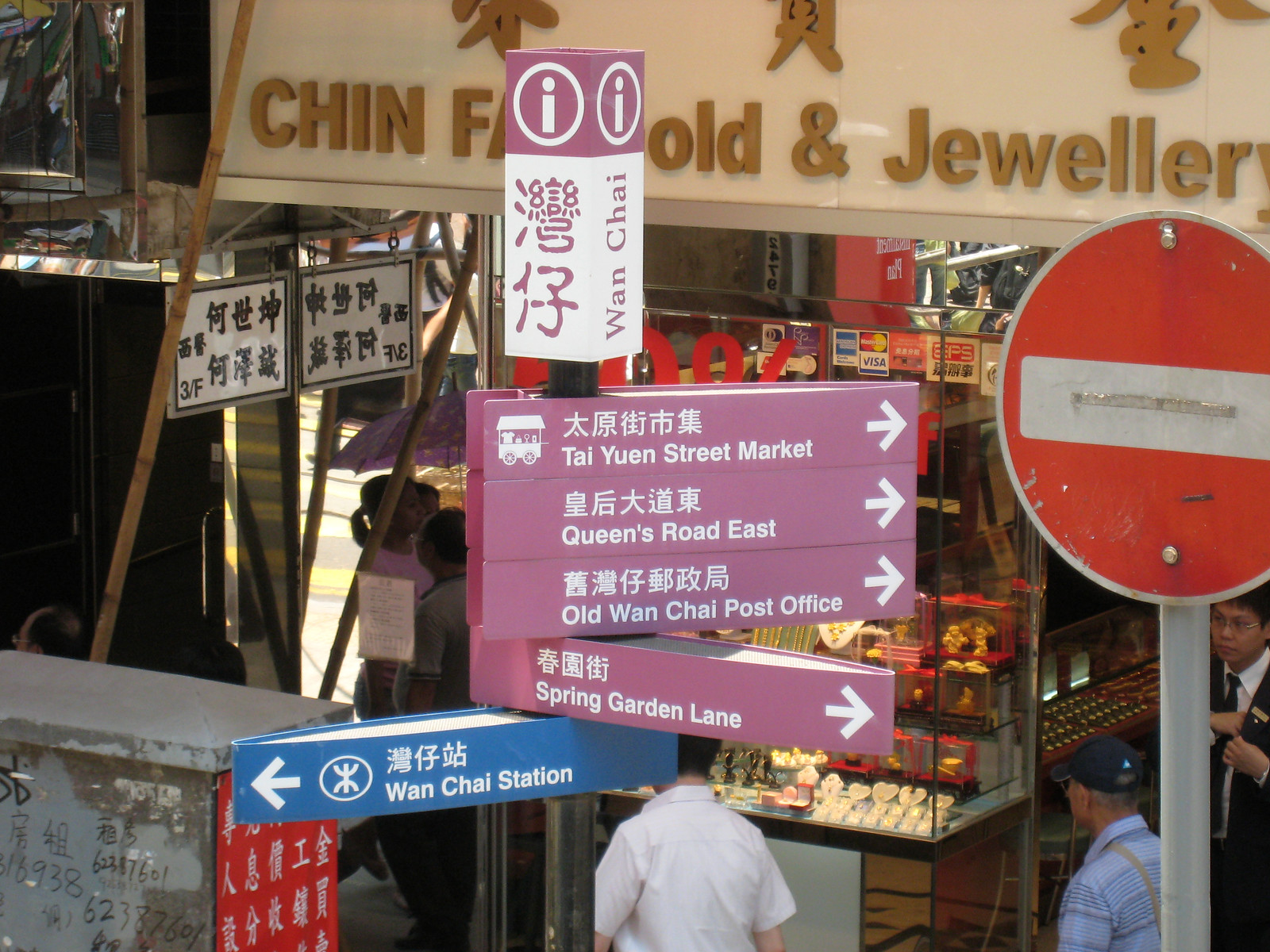In the image, there's a busy scene at a bustling health area in Hong Kong. Prominently featured is an informative signpost with a purple box at the top containing a white circle and the letter "I" for information. To its left, there are Chinese characters, and the right side reads "Wan Chai." Below this, the signpost is divided into four sections with the same purple backdrop. The first three point to the right: "Tai Yin Street Market," "Queens Road East," and "Old Wan Chai Post Office," each with respective arrows. The fourth section, slightly tilted, points the way to "Spring Garden Lane." Additionally, at the bottom of the sign, a blue section directs towards "Wan Chai Station" with an arrow to the left. To the right, there's a traffic sign with an orange background and a white rectangle, mounted on a silver post. The background reveals a white billboard with partial gold lettering, visible as "Jin F... Old and Jewelry," hinting at a jewelry shop nearby. The area is bustling with people, likely exploring the various attractions and shopping options available.